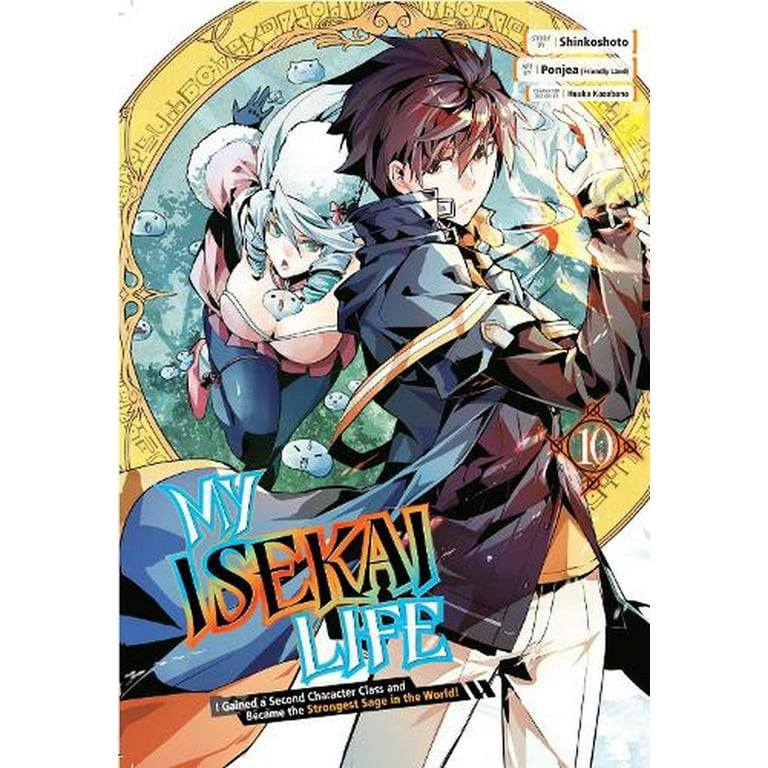A vibrant, vertically aligned rectangular image presents a dynamic anime poster without a border. Dominating the center is a young boy with spiky brown hair, shown from his right side, dressed in a tan and brown jacket, white pants, and a belt or sash tied around his waist. His body faces slightly backward with his head turned forward, adding a sense of motion. The background features a large, dull gold circular object resembling a coin or portal, containing additional anime figures, including a girl with gray, poofy hair styled in swirly ponytails. She wears a pink top and blue pants, bent forward as if running towards the boy. In the lower left, block style letters spell out "My Isekai Life" with "My" and "Life" in white with blue outlines, and "Isekai" in black with a yellow and orange border. At the very bottom, bold text announces, "I gained a second character class and became the strongest sage in the world!"